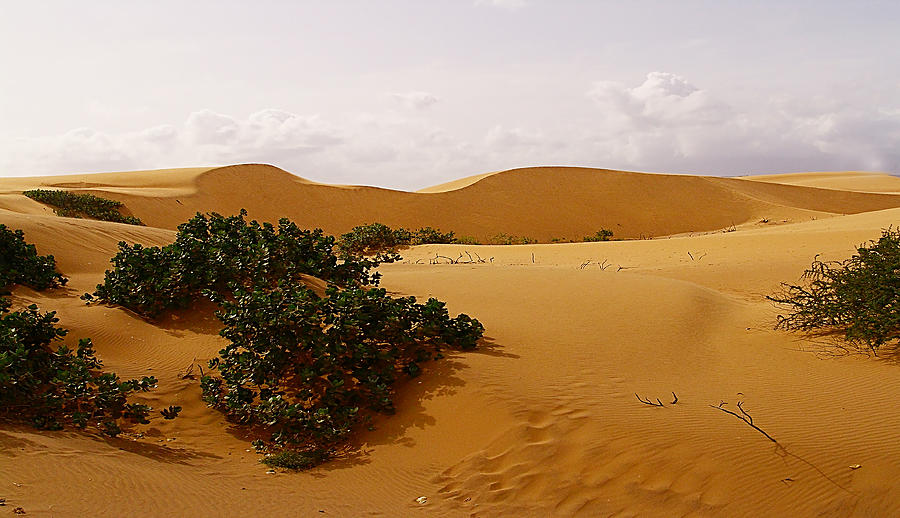The image features a barren desert landscape dominated by rolling sand dunes of a bright mustard-yellow and orange hue. These undulating dunes are punctuated by scattered bushes, primarily small, ground-cover shrubs, and occasional protruding branches partially buried in the sand. The sky, which occupies about half of the frame, is overcast and devoid of blue, presenting layers of dark, hazy clouds that contribute to the overall dim lighting of the scene. Remarkable details include faint, possibly wind-sculpted patterns on the dunes, slight greenery at certain spots, and indistinct animal footprints on the right side of the image, adding a subtle touch of life to this otherwise desolate panorama.